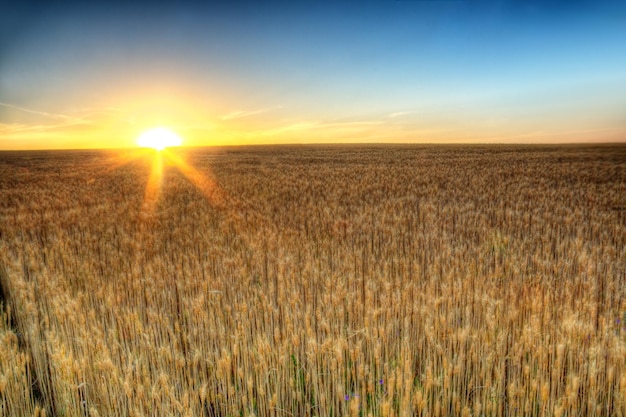This image captures a vast, flat wheat field extending to the horizon, with stalks standing straight and topped with small golden seed heads that have a soft, almost cottony appearance. The wheat is a golden color, with a hint of green at the bottom of the stems. In the top left corner, the Sun is either rising or setting, positioned halfway above the horizon. The Sun emits a bright white light at its core that transitions into yellow and pink hues, eventually blending into a violet ambiance with a dark blue sky at the very top. The sky is primarily blue, speckled with a few clouds that catch the sunlight, sending beams across the field and creating a soft glow. A subtle pathway can be faintly seen in the lower left corner, with some tiny violet flowers and a few green plants adding slight variations to the otherwise endless sea of golden wheat.